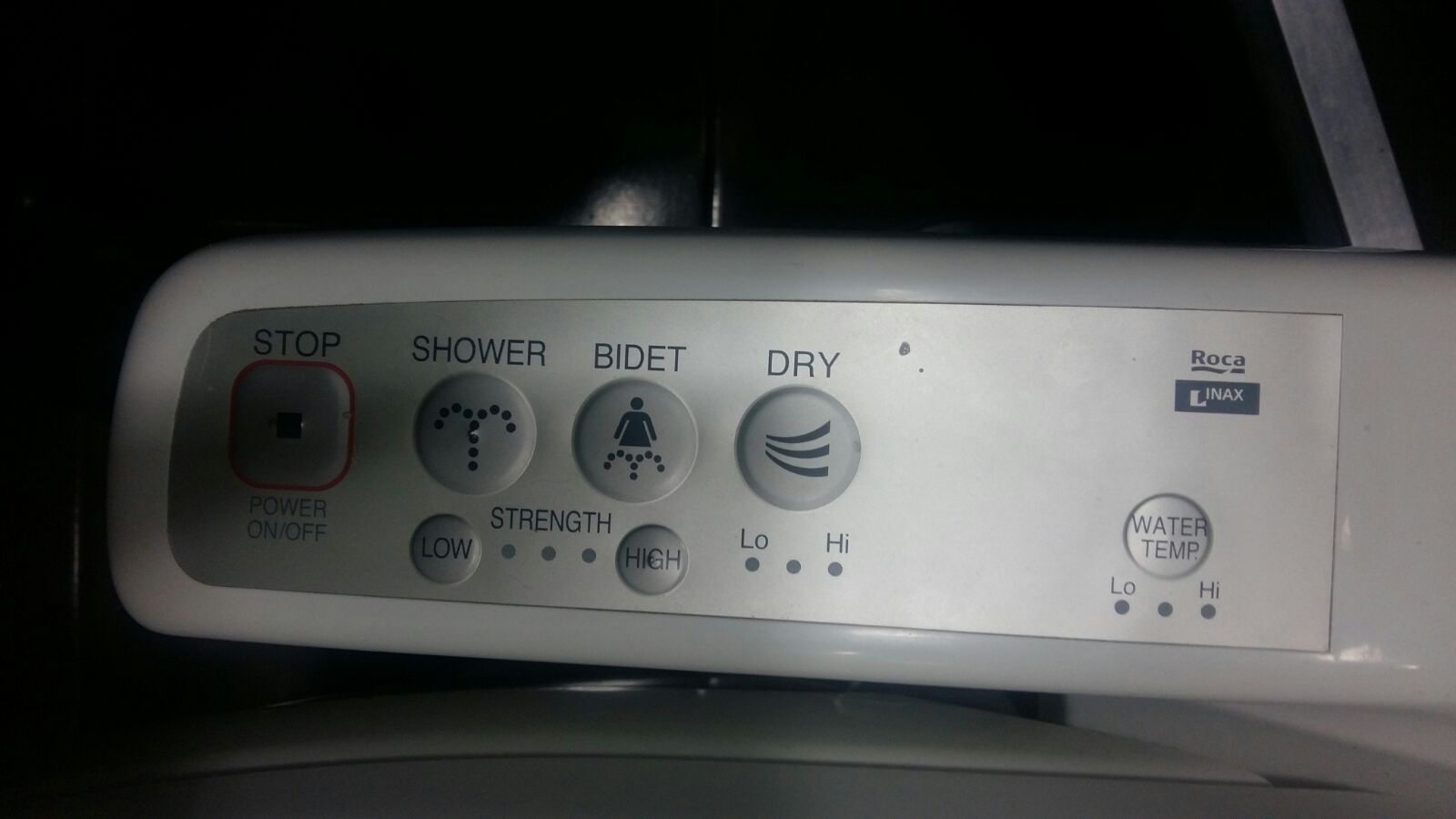This image showcases a white control device, likely for a toilet, bidet, or integrated shower system, positioned centrally against a predominantly dark background, suggesting it was taken in a dimly lit or nighttime indoor setting, possibly a bathroom. The device features several labeled buttons: a prominent "STOP" button with a red border, alongside "SHOWER," "BIDET," and "DRY" buttons. Below these, there are controls for adjusting the strength from "LOW" to "HIGH" and a "WATER TEMP" button to the right. The background is almost entirely black, adding to the emphasis on the white and light gray tones of the control unit, which is vividly illuminated by a subtle light source. The image is composed primarily of black, white, gray, red, and hints of dark blue, underscoring the technical and modern aesthetic of the remote-like device.